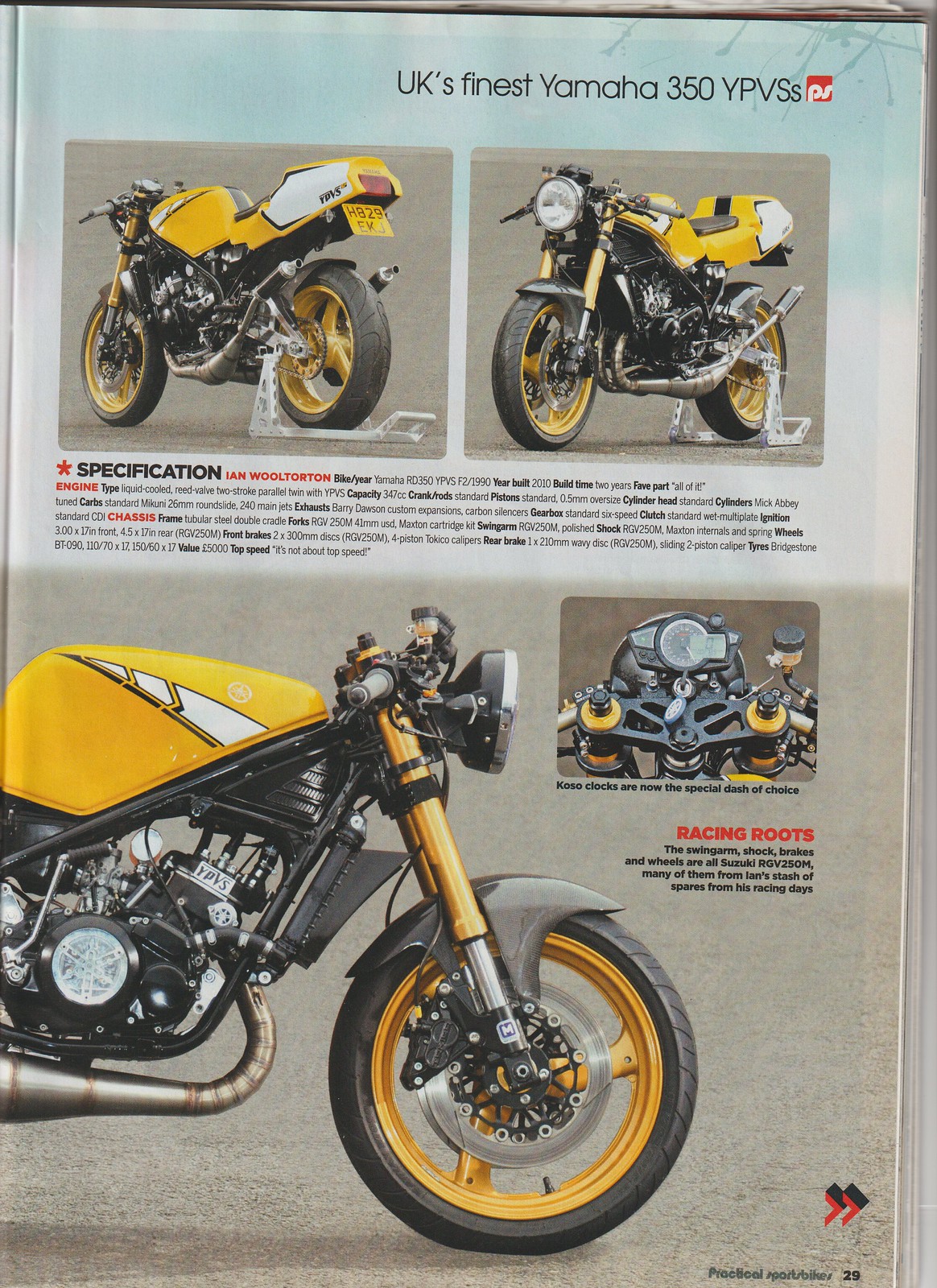The image is an advertisement for the UK's finest Yamaha 350 YPVS-S, featured on page 29 of a magazine. The layout includes four distinct shots of the yellow and black street motorcycle, complemented by detailed but unreadable specification text. In the upper left, there is a rear-left quarter shot at a 45-degree angle, while the upper right exhibits a front-right 45-degree angle view. Dominating the lower half of the page is an extensive forward right-side shot, revealing the gas tank, front wheel, and the addition of disc brakes. Adjacent is a smaller inset highlighting the cockpit with Koso clocks as the special dash choice. The text emphasizes the motorcycle’s high-performance features, such as its Suzuki RGV250M swingarm, shock, brakes, and wheels, sourced from Ian Wool-Torton’s racing parts stash. The background of the image suggests it was taken from a physical magazine, evoking a concrete or road surface backdrop and a distinctive white and blue design in the top third.